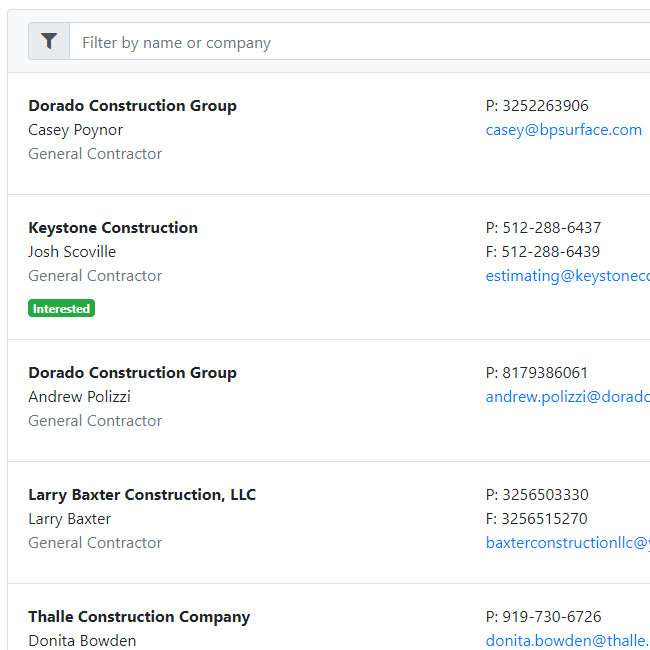The image displays a list of general contractors with their contact information, organized in a structured format. At the top of the page, there is a small search bar labeled "Filter by name or company."

- **Dorado Construction Group**
  - KC, Poynort General Contractor
  - Phone: P3252263906
  - Email: kc@bpservice.com (in blue text)

- **Keystone Construction**
  - Josh Scoville, General Contractor
  - Green banner with white text stating "Interested"
  - Phone: 512-288-6437
  - Text: 512-288-6439
  - Email: estimate@keystoneconstruction.com

- **Dorado Construction Group**
  - Andrew Polizzi, General Contractor
  - Phone: 817-938-6061
  - Email: andrew.polizzi@doradoconstruction.com

- **Larry Baxter Constructions LLC**
  - Larry Baxter, General Contractor
  - Phone: 325-650-3330
  - Fax: 325-651-5270